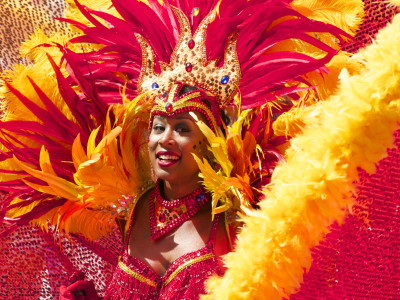In the vivid photograph, a woman is the focal point, adorned in elaborate and flamboyant attire suggestive of a carnival or festival theme. From the chest upwards, she is wearing a striking red and yellow outfit that almost takes up the entire frame. The outfit features feather-like structures, radiating outwards like expansive wings, with red at the center and yellow along the outer edges, lavishly decorated with sequins of red, yellow, and a hint of blue. Her neck piece is a thick, V-shaped collar with sequins mirroring the outfit’s vibrant colors.

She sports vivid makeup, including red lipstick and blue and yellow cheek markings. Her headpiece is particularly elaborate—it resembles a crown or headdress with red and gold components, resembling flaming emanations. This headdress is adorned with sparkling gems: red rubies and blue stones, with one ruby-like gem centered on her forehead and additional blue stones on either side. To accentuate the grandiosity, the headdress is tufted with pink feathers behind her head, creating an impression of fiery exuberance.